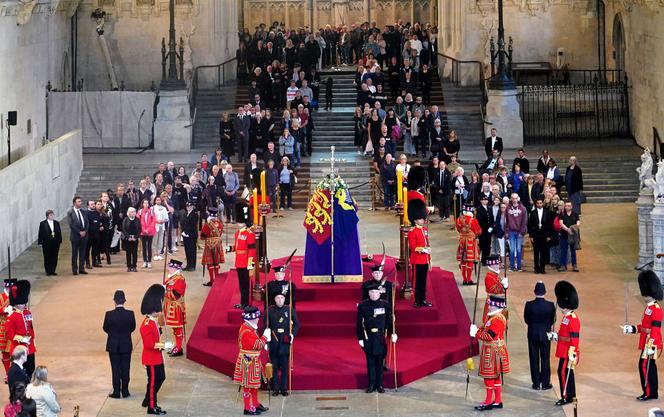In the image, we witness a grand royal ceremony taking place within the stately confines of a throne room or grand public ceremony hall. At the center of the room is a burgundy riser, prominently placed as the focal point of the event, surrounded by an array of people. The riser supports a casket draped in a ceremonial cloth of blue, red, and yellow. Encircling the riser are two sets of guards: one group in distinct red uniforms, black pants, and tall black bearskin hats positioned at each corner, while another set of guards, clad entirely in black uniforms with ornate feathers on their caps, stands immediately around the casket, holding golden staffs.

The room itself is constructed with imposing gray granite walls adorned with statuary resembling gargoyles, adding to the grandeur and solemnity of the occasion. Behind the central platform, a multitude of formally dressed witnesses gather, filling the stairways that lead up to a large, ornately crafted door, likely the entrance to a palace. The layout suggests a momentous event—possibly a coronation or a royal procession. Attendees seem to pay their respects to a high-ranking royal figure, reflecting the solemn and regal nature of the ceremony.